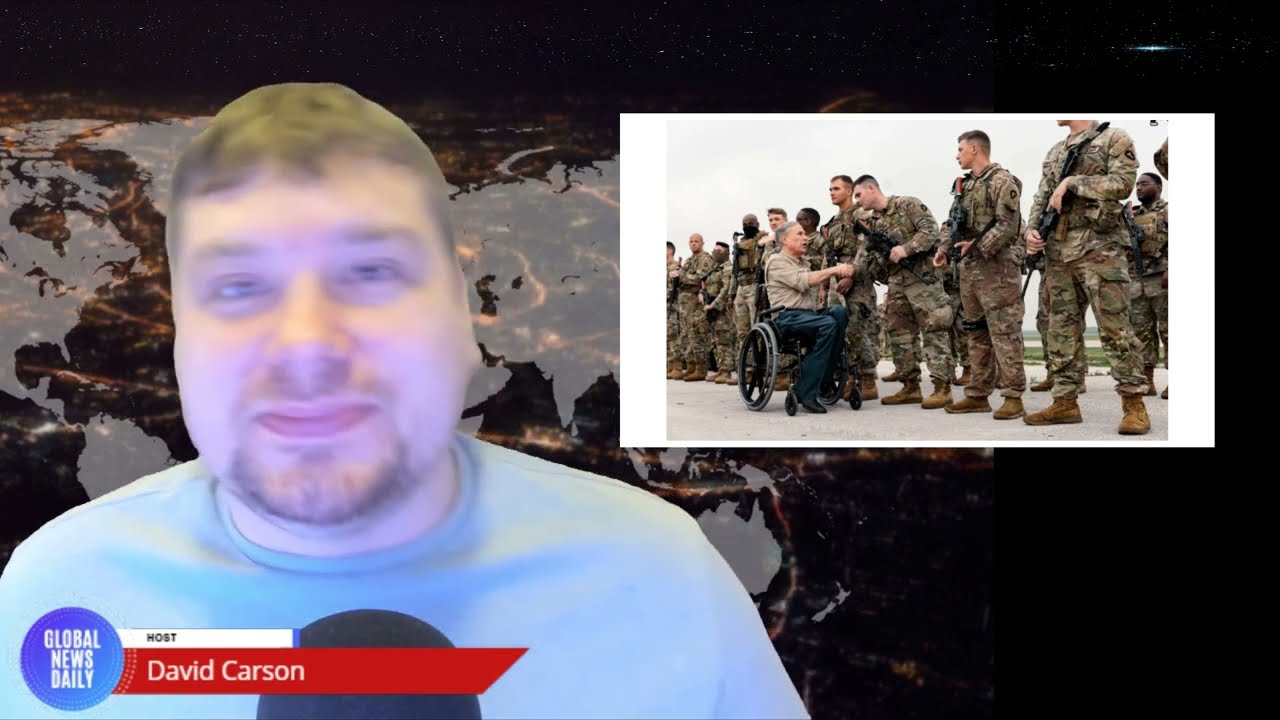In this image, a man is presenting a newscast for 'Global News Daily.' The host, identified as David Carson by an on-screen label, is a Caucasian male with short brown hair, a short goatee, and a beard. He is wearing a light blue shirt and speaking into a microphone. Behind him is a green screen displaying a globe against a black background dotted with stars. In the upper right-hand corner of the screen, there is a photograph depicting several soldiers in military uniforms standing in a line on a grass field. In this image, one soldier is seen shaking hands with a veteran in a wheelchair who is dressed in blue pants and a gray jacket under a white sky.